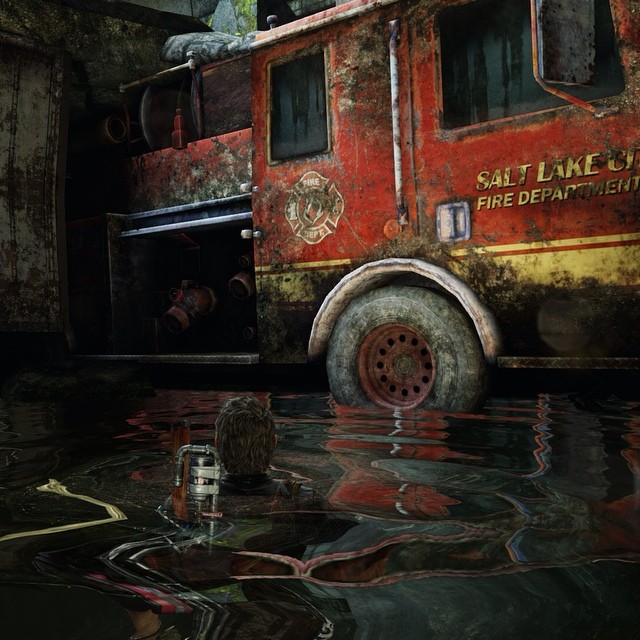In the foreground of this image, a body of water creates a smooth, rippling surface. At the bottom, an individual is partially submerged, wearing a scuba tank visible from the shoulders upward. The top of the scuba tank is apparent just above the waterline, adding to the scene's intrigue.

Rising from the middle to the top of the picture stands a weathered and extremely beat-up Salt Lake City Fire Department fire truck. The truck is significantly rusted, with dirt-encrusted tires that suggest prolonged exposure to harsh conditions. One of the storage compartments on the truck is open, revealing various pieces of firefighting equipment. The rear of the truck is not fully visible, suggesting that the vehicle extends beyond the right edge of the image.

Overall, this detailed scene highlights the juxtaposition of aquatic rescue readiness against the backdrop of a heavily used and timeworn emergency vehicle.